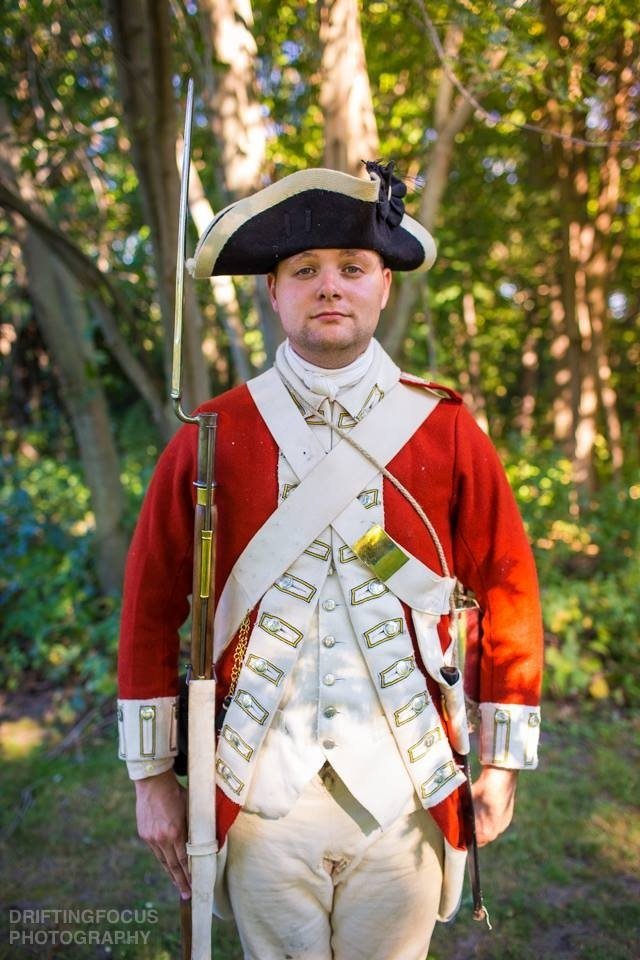In this detailed portrait, a man dressed as a British redcoat from the Revolutionary War era poses facing directly at the camera. He wears an authentically styled uniform that includes a striking red coat adorned with gold buttons and white cross straps that form an X over his chest. Underneath, he has a white vest and white pants. On his head rests a distinctive tricorn hat, black with gold trim, which is slightly tilted, adding to the historical accuracy of his attire. In his right hand, he firmly grasps a musket fitted with a bayonet at the end. The musket itself features a white body with a wooden section around the muzzle. He stands confidently on a grassy patch, surrounded by a background of lush green trees and bushes. The image bears a watermark in the bottom left corner reading "Drifting Focus Photography," marking its artistry and origin.